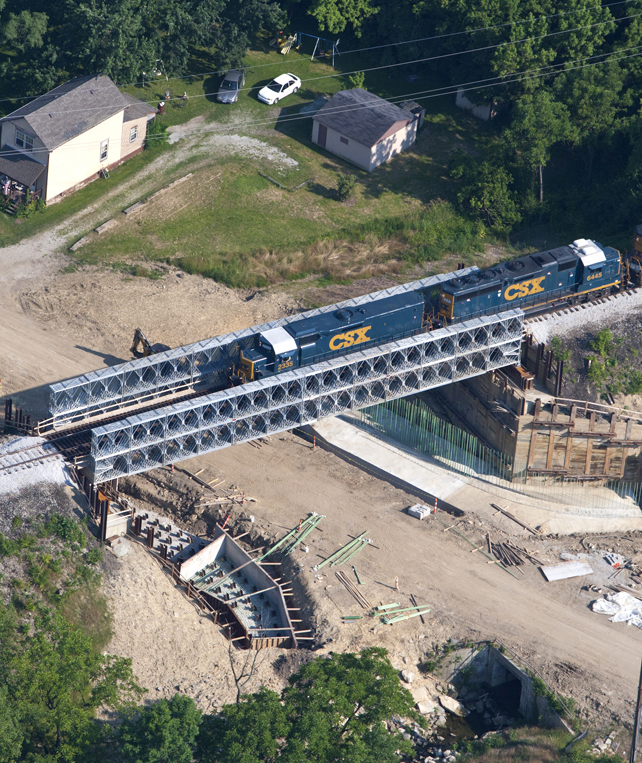The image captures an aerial view of a partially constructed metal railway bridge, prominently featuring a CSX train in transit. The bridge spans a dirt underpass, and its latticework of steel offers an unfinished look, as materials scattered around hint at ongoing construction. Unusually, two blue cabooses with yellow writing are linked together, devoid of any connecting cars, and contrasting the described rich forest green engine in other accounts. Both elements bear the distinctive orange "CSX" lettering. In the backdrop, two white houses - one larger and one smaller - stand close to the tracks, with a white and a gray car parked on the green grass between them. The surrounding environment includes grass, trees, and bushes, enhancing the picturesque setting on this sunny day.